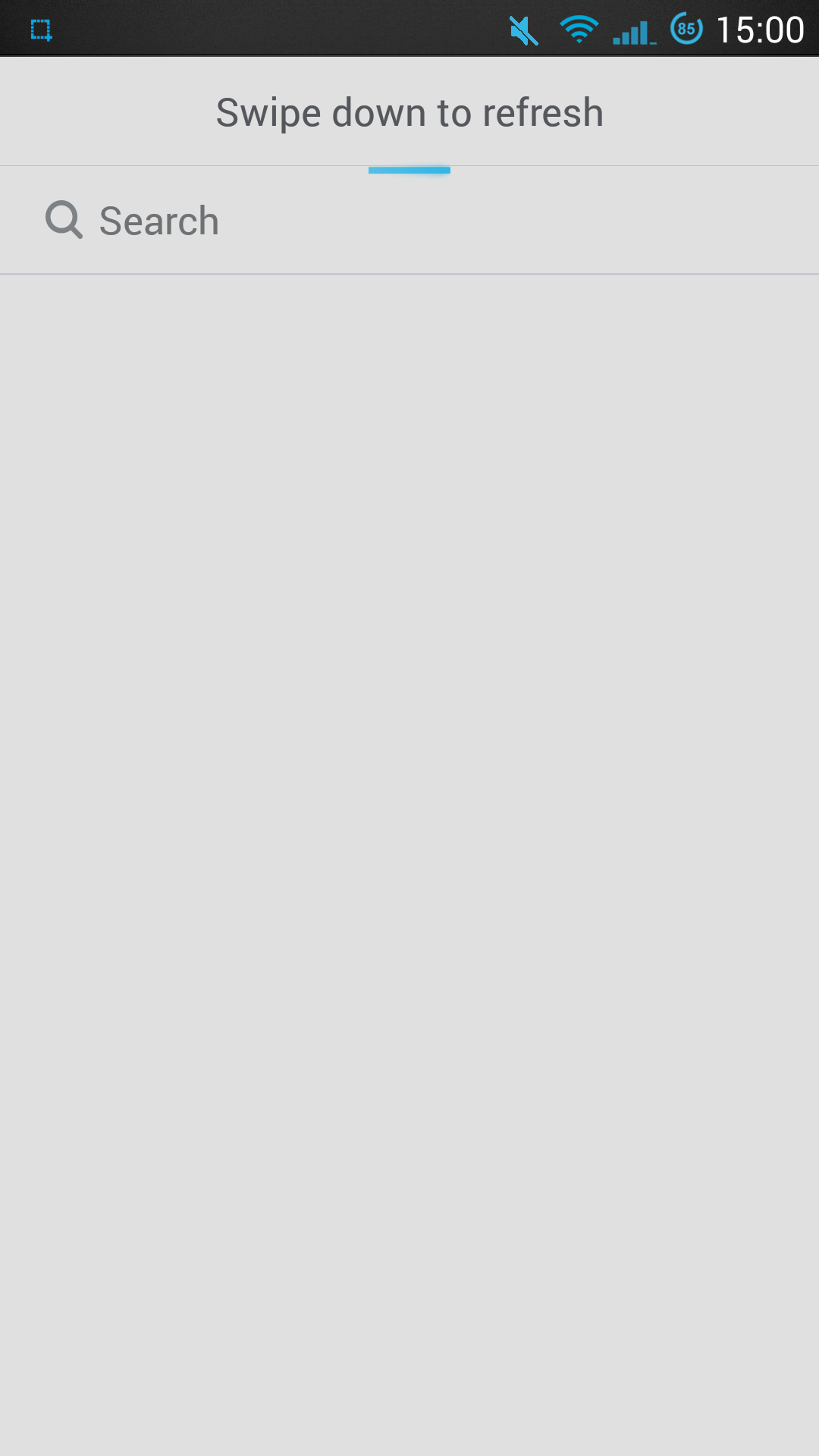The top left corner of the screen displays a blue square with a speaker icon that has a slash through it, indicating that the sound is muted. The Wi-Fi signal is nearly full, with only one bar missing. The battery level is at 85%. Adjacent to these icons, white text reads "15" over a gray background, likely the current time. There is a prompt to "Slide down to refresh" and a search bar available. The black bar at the very top of the screen houses these icons and indicators. Overall, the screen is primarily gray with minimal lines and text, representing a typical smartphone interface with muted sound and active internet connectivity.